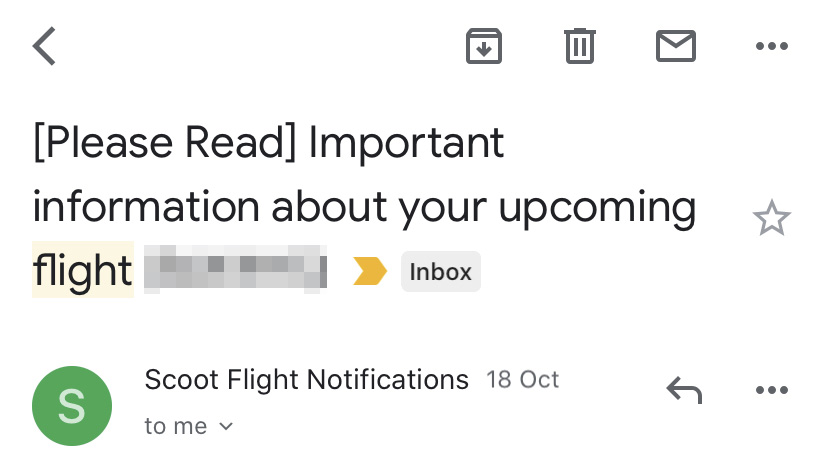This is a detailed and meticulous description of an email screenshot captured from Google Mail. 

At the top right corner of the screenshot, there are three icons: a trash bin, a mail envelope, and an ellipsis (three vertical dots). The subject line of the email, written in black text, reads: "Important Information About Your Upcoming Flight," with the phrase "please read" enclosed in brackets. Notably, the word "Flight" is highlighted in yellow, while the word immediately following it has been redacted and blurred out. 

A thick yellow arrow points towards the right, aiming at a gray box labeled "Inbox." On the far right of this line, there is a star icon. 

Underneath the subject line, there is an avatar – a green circle with the letter "S" emblazoned on it. To the right of this avatar is the sender's information: "Scoot Flight Notifications for 18 of October," followed by a downward-pointing arrow indicating a dropdown menu. 

On the far right side of the screen are a back button (a leftward-pointing arrow) and another ellipsis (three vertical dots).

This thorough description captures all significant details and provides a vivid visualization of the email screenshot.